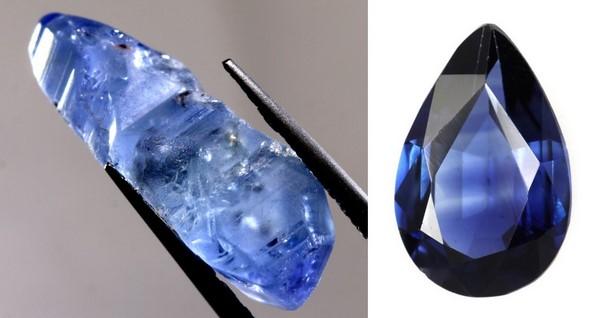The paired images showcase an intricate and vivid display of what appears to be the evolution of a blue gemstone. In the first image, a set of black, needle-nosed tweezers gently holds a roughly hewn blue crystal with ocean blue and white blended hues. This raw crystal is illuminated against a light gray background, highlighting its varying opacity and vibrant, reflective surfaces. Adjacent to this, the second image displays the same type of gem, now meticulously polished and cut into an oval teardrop shape with well-defined facets. This finished gem, resembling the deep blue of a sapphire, is clearer and glossier, set against a dark gray background. This juxtaposition beautifully contrasts the natural, unrefined state of the gemstone with its potential as a refined, jewelry-worthy artifact.